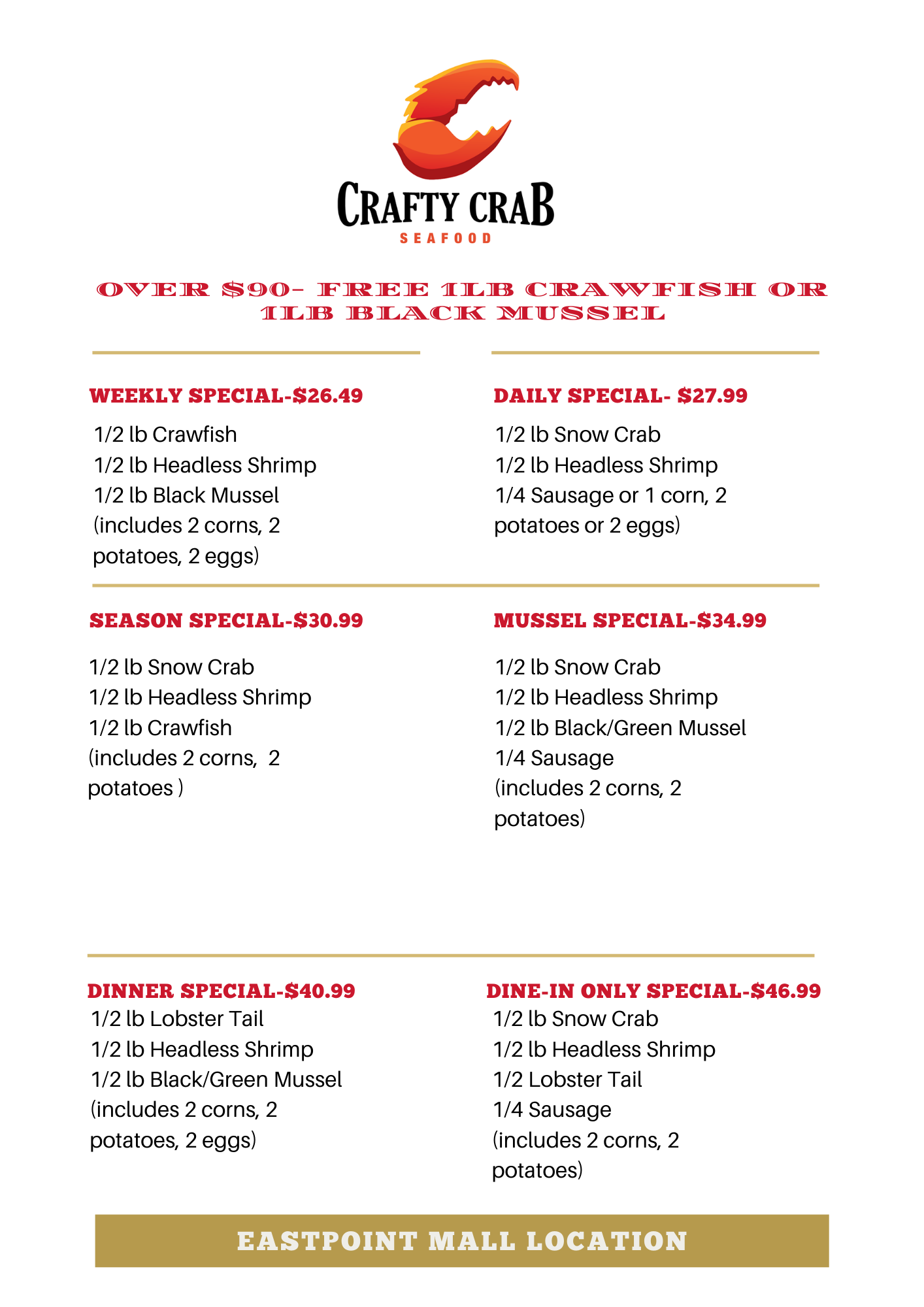This is a detailed menu listing for Crafty Crab Seafood Restaurant, prominently featuring a crab claw logo at the top. Below the logo, the name "Crafty Crab Seafood" is displayed, with “Crafty Crab” in black letters and “Seafood” in red. The menu is from the East Point Mall location.

At the top, there is a promotion stating that any purchase over $90 earns a free pound of crawfish or black mussels. The menu is divided into several sections, each with a special seafood combo:

1. **Weekly Special - $26.49**: Includes 1 lb. crawfish, 1 lb. headless shrimp, and 1 lb. black mussel, served with 2 corns, 2 potatoes, and 2 eggs.
2. **Daily Special - $27.99**: Features 1 lb. snow crab, 1 lb. headless shrimp, and a choice of either 1 lb. sausage or 1 corn, as well as 2 potatoes or 2 eggs.
3. **Season Special - $30.99**: Contains 1 lb. snow crab, 1 lb. headless shrimp, and 1 lb. crawfish, including 2 corns and 2 potatoes.
4. **Mussel Special - $34.99**: Offers 1 lb. snow crab, 1 lb. headless shrimp, and 1 lb. black and green mussels, plus 1 lb. sausage, 2 corns, and 2 potatoes.
5. **Dinner Special - $40.99**: Consists of 1 lb. lobster tail, 1 lb. headless shrimp, and 1 lb. green and black mussels, accompanied by 2 corns, 2 potatoes, and 2 eggs.
6. **Dine-In Only Special - $46.99**: Includes 1 lb. snow crab, 1 lb. headless shrimp, 1 lb. lobster tail, and 1 lb. sausage, along with 2 corns and 2 potatoes.

Each special is clearly outlined, making it easy for patrons to choose their preferred seafood combination. The beige background and white lettering at the bottom emphasizing the East Point Mall location add a clean and professional touch to the menu.